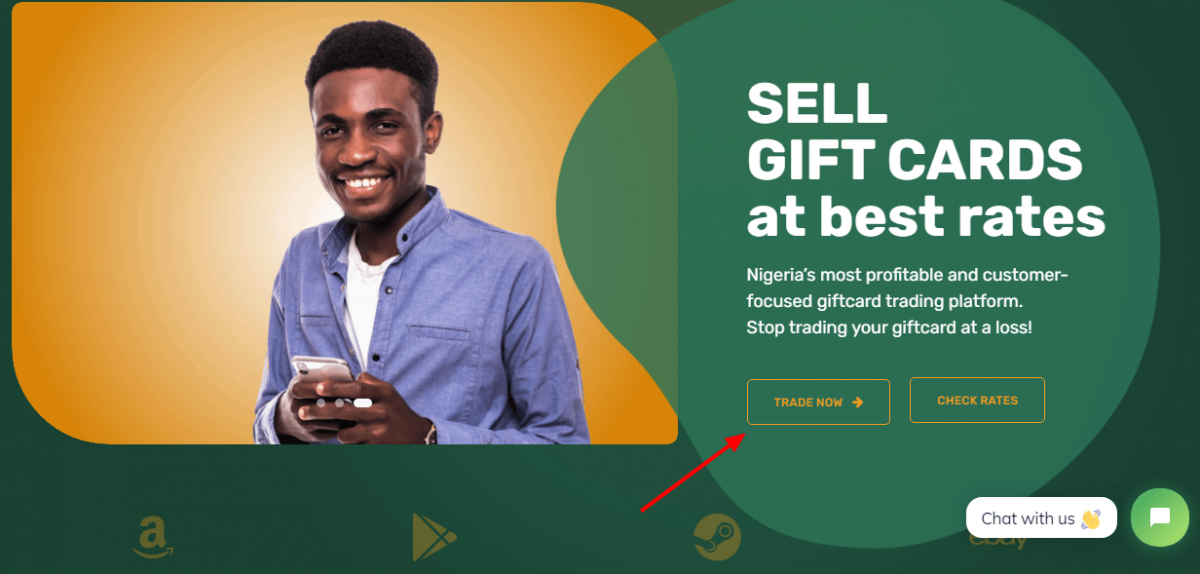The image depicts a screenshot of a website featuring a vibrant green background. The layout is a horizontal rectangle, with a significant segment on the upper left side dominated by a yellow, almost-rectangular shape with rounded corners. Within this yellow area, there is a photograph of a smiling black man with short hair on the sides and slightly longer hair on top. He is dressed in a long, blue button-down shirt with a white undershirt and is holding a cell phone in front of him.

To the right of the man, there is a blob-like, non-circular shape in a lighter shade of green. This shape contains white text promoting the website's services: "Sell gift cards at best rates. Nigeria's most profitable and customer-focused gift card trading platform. Stop trading your gift card at a loss." Below this text are two clickable buttons labeled "Trade Now" and "Check Rates." A prominent red arrow starts from the bottom center of the image, pointing diagonally upward towards the "Trade Now" button, drawing attention to it.

In the bottom right corner, there is a large white oval with the text "Chat with us." Inside the oval is an image of a yellow figure or object. To the immediate right of this oval is a green circular chat button featuring a word bubble icon, indicating an option for live chat support.